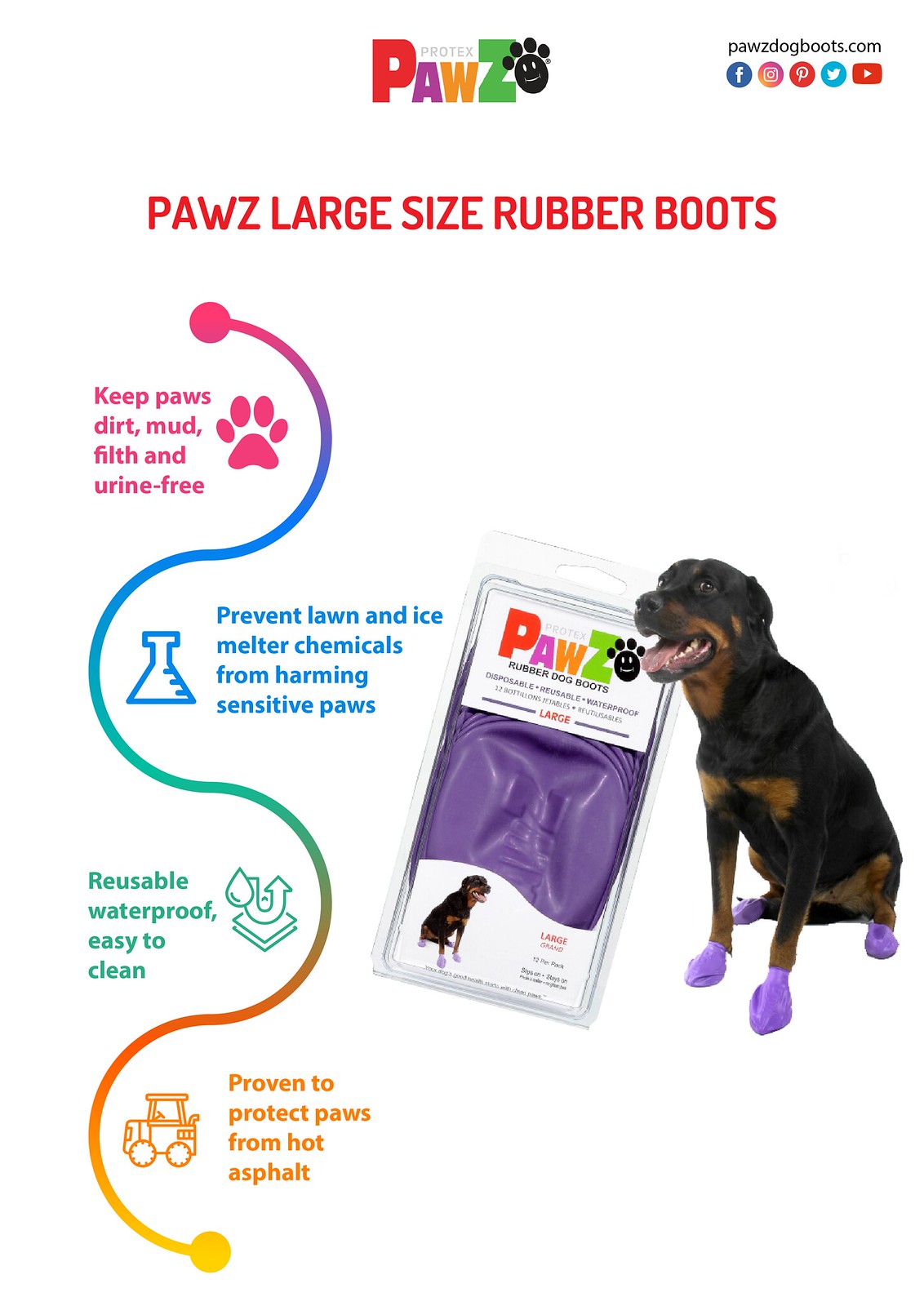The image is a detailed advertisement for a canine product called "PROTEXPAWZ," showcasing protective rubber boots for dogs. Set against a predominantly white background, the central focus is a medium-sized black and brown dog, possibly a Rottweiler or Doberman, sitting and wearing purple rubber boots, described as "PAWZ." To the left side of the dog is a package of the same product, featuring a mirrored image of the dog on the bottom left corner. The package displays the brand name "PAWZ" in large text with distinct multi-colored letters: the P is red, the A is purple, the W is orange, and the Z is green. The top header of the package is red and reads "Large Size Rubber Boots."

A vertical, multi-colored wavy line runs along the left side of the image, beside which four bullet points list the product's features: keeping paws free from dirt, mud, filth, and urine; preventing damage from lawn and ice melter chemicals; being reusable, waterproof, and easy to clean; and offering protection against hot asphalt. The boxed product itself is displayed with the same colorful "PAWZ" logo and includes additional descriptors as one moves down the label. In the top right corner of the advertisement, a URL and social media icons are also visible. The overall presentation emphasizes the product's functionality and protective benefits for dogs, making it both appealing and informative.